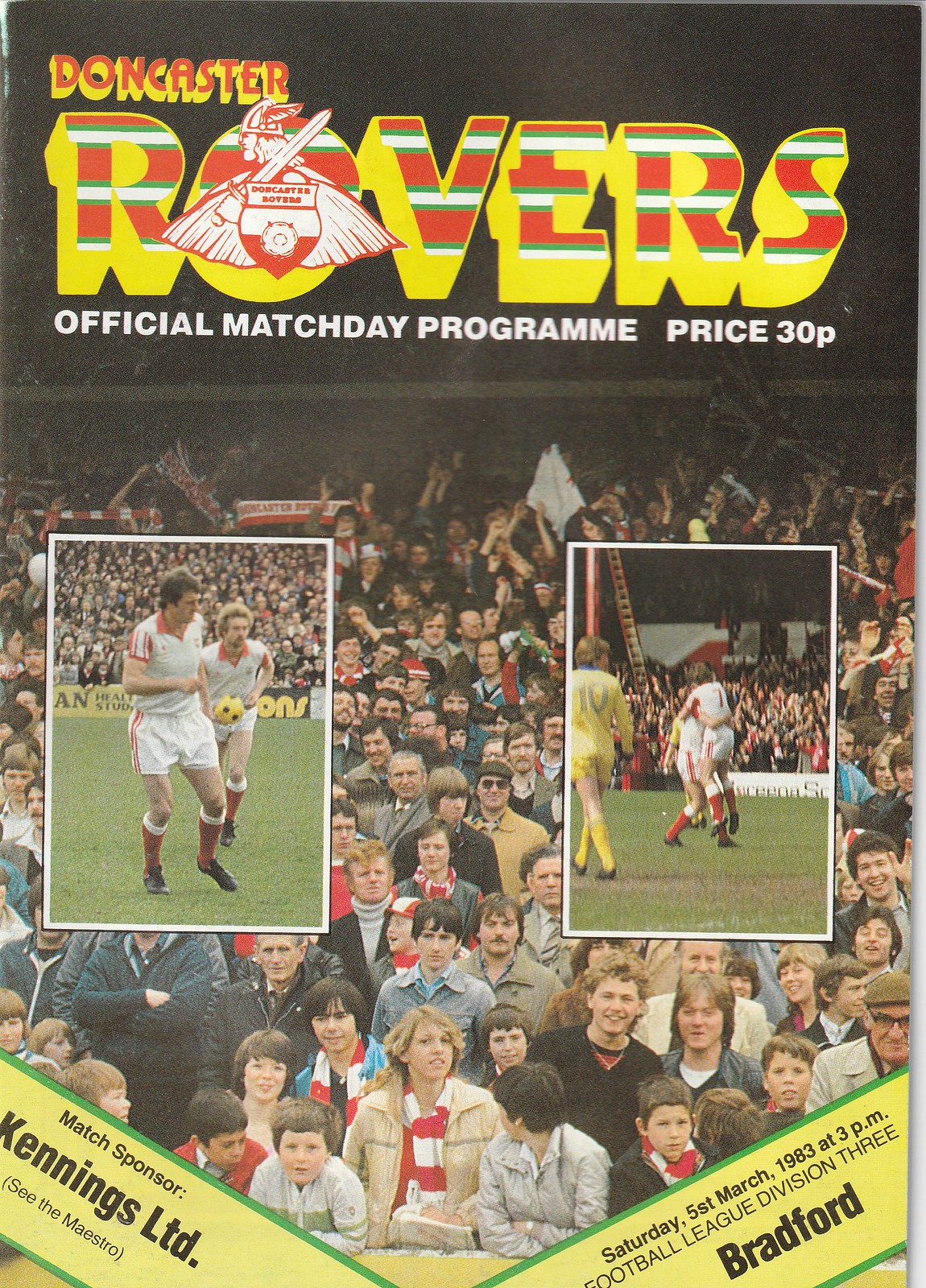The front page of the Official Match Day Program for the Downeaster Rovers, priced at 30 pence, features a vibrant and detailed design. At the top, "Doncaster Rovers" is prominently displayed in yellow and red letters, accented with horizontal blue and white stripes. The "O" in "Rovers" is cleverly replaced with a rover symbol—depicting a knight holding a sword—against a nearly black background.

Beneath this header, the text reads "Official Match Day Program" in white print. The lower two-thirds of the cover showcases an engaging photo of cheering soccer fans in the stands, all enjoying what appears to be a pleasant day. Superimposed on this crowd image are two inset photos of players. The left inset shows two players in white jerseys, white shorts, red socks, and black cleats, contending for a yellow soccer ball with black accents. The right inset features the same players embracing, celebrating a moment on the pitch. 

Adding to the dynamic layout are two diagonal yellow banners with green borders positioned along the bottom. The left banner announces "Match Sponsor: Kenningtons Limited," and the right one provides the match details: "Saturday, 5th March 1983 at 3 p.m. Football League Division III, Bradford." The overall effect is a lively and celebratory cover that captures the excitement and detail of match day.